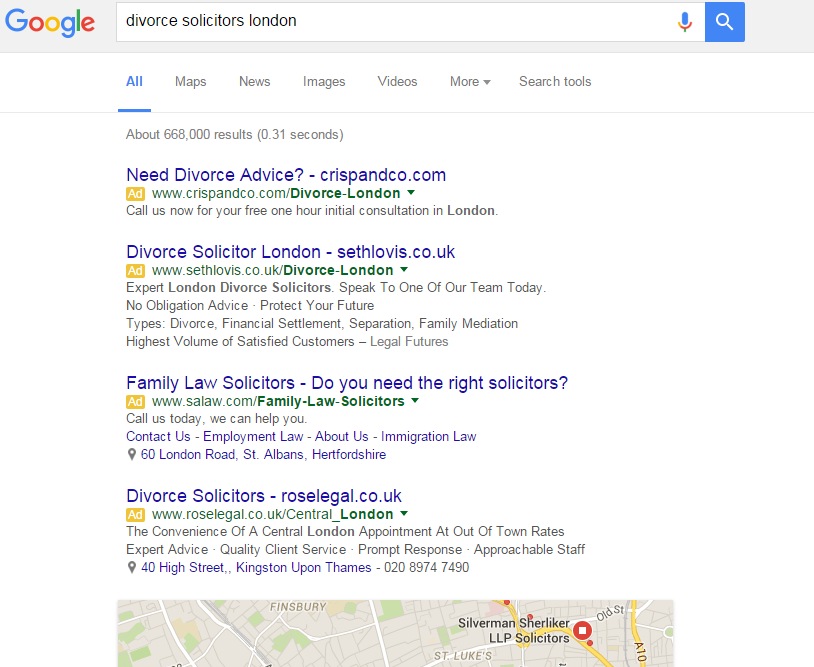**Screenshot Description: Google Search for "Divorce Solicitors London"**

The image depicts a screenshot of a Google search results page. At the top of the screen, the iconic Google logo is visible, with the capital 'G' in blue, followed by the 'o's in red and yellow, the lowercase 'g' in blue, 'l' in green, and 'e' in red again. 

Below the logo is the search bar, which contains the query "divorce solicitors London". To the right of the search bar, there are two icons: a microphone icon for voice search and a magnifying glass icon for initiating the search, both inside a blue outlined square.

Directly beneath the search bar is a horizontal menu with several options including "All," "Maps," "News," "Images," "Videos," and "More." The "All" option is underlined in blue, indicating that it is the selected tab. To the right of these options is a link labeled "Search tools."

The search results section begins with a note indicating that there are approximately 668,000 results, generated in 0.31 seconds.

The first few listings are marked as sponsored ads. The top result has a title "Need Divorce Advice - Chris C.r.i.s.p.n.p.n.d.c.o.com" with an 'Ad' label in yellow next to it. Following this, there's another sponsored result titled "Divorce Solicitor London - S.e.t.h.l.o.v.i.s.co.uk."

Subsequent to these ads, the search results include links to various solicitor firms:
1. "Family Law Solicitors – ‘Do You Have the Right Solicitors?’" 
2. "Divorce Solicitors – RoseLegal.co.uk"

At the bottom of the screenshot, there is a partial view of a map highlighting local solicitors with a listing for "Silver & Sure Lekker LLP Solicitors."

Overall, the screenshot captures an organized display of search engine results for individuals seeking divorce solicitors in London.